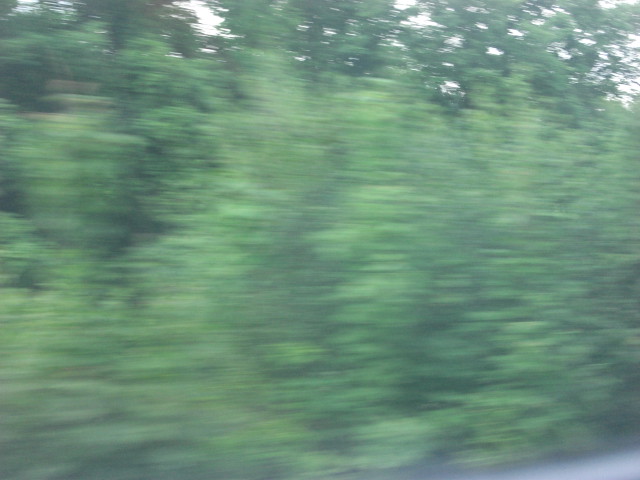The image depicts a blurred view of lush green foliage, suggesting it was captured in motion, possibly from a moving car. The greenery consists mainly of dense bushes and lighter green vegetation, which cover about 95% of the image. In the upper portion, especially on the right side, there are treetops with slightly less blurring, contrasting with the darker, different types of trees toward the top one-third. Small gaps between the foliage reveal hints of a cloudy sky with some faint blue patches. At the bottom right corner, a small strip of gray, likely a road with white curb paint, is barely noticeable. Overall, the image, taken during the daytime, conveys a sense of rapid movement through a green, natural landscape.